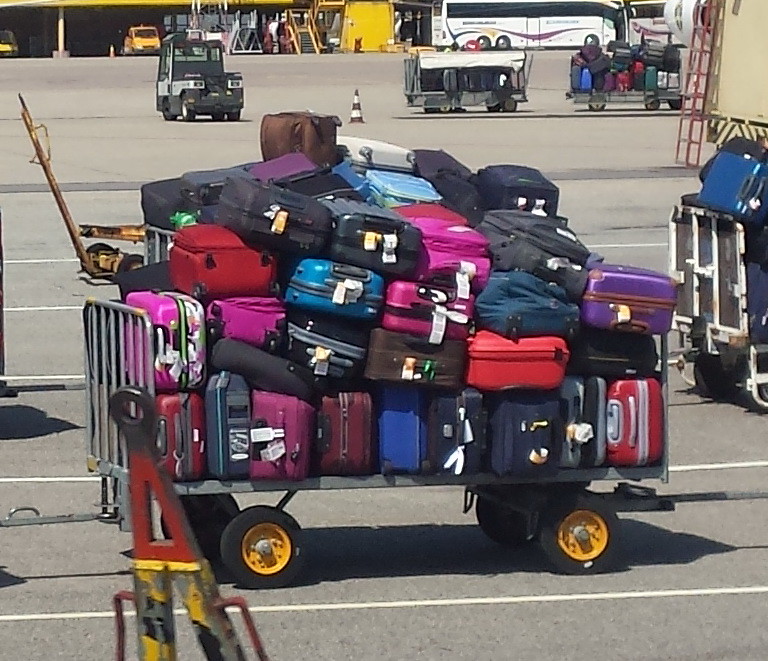This image is an outdoor scene, likely at an airport, showcasing a large metal baggage cart with four wheels, piled high with a diverse array of colorful luggage. The cart holds suitcases in shades of pink, red, blue, maroon, purple, gray, brown, and the ubiquitous black, all adorned with destination tags wrapped around their handles. The neatly arranged bottom layer contrasts with the more randomly stacked suitcases on top. Behind this cart, another partially visible cart, also filled with luggage, is hooked to it. 

Further in the background, the setting includes several motorized carts that are likely used by airport staff to transport luggage, a bus for tour groups, and an open garage with a yellow vehicle and other equipment. The scene is set on a gray pavement marked with white lines, suggesting an organized yet bustling environment where luggage is presumably being prepared for loading onto airplanes. The foreground features a red triangular object, possibly part of the equipment used to maneuver the carts. This busy and vibrant image captures the dynamic backstage operations at an airport, showcasing the logistics of handling numerous suitcases and preparing them for travel.